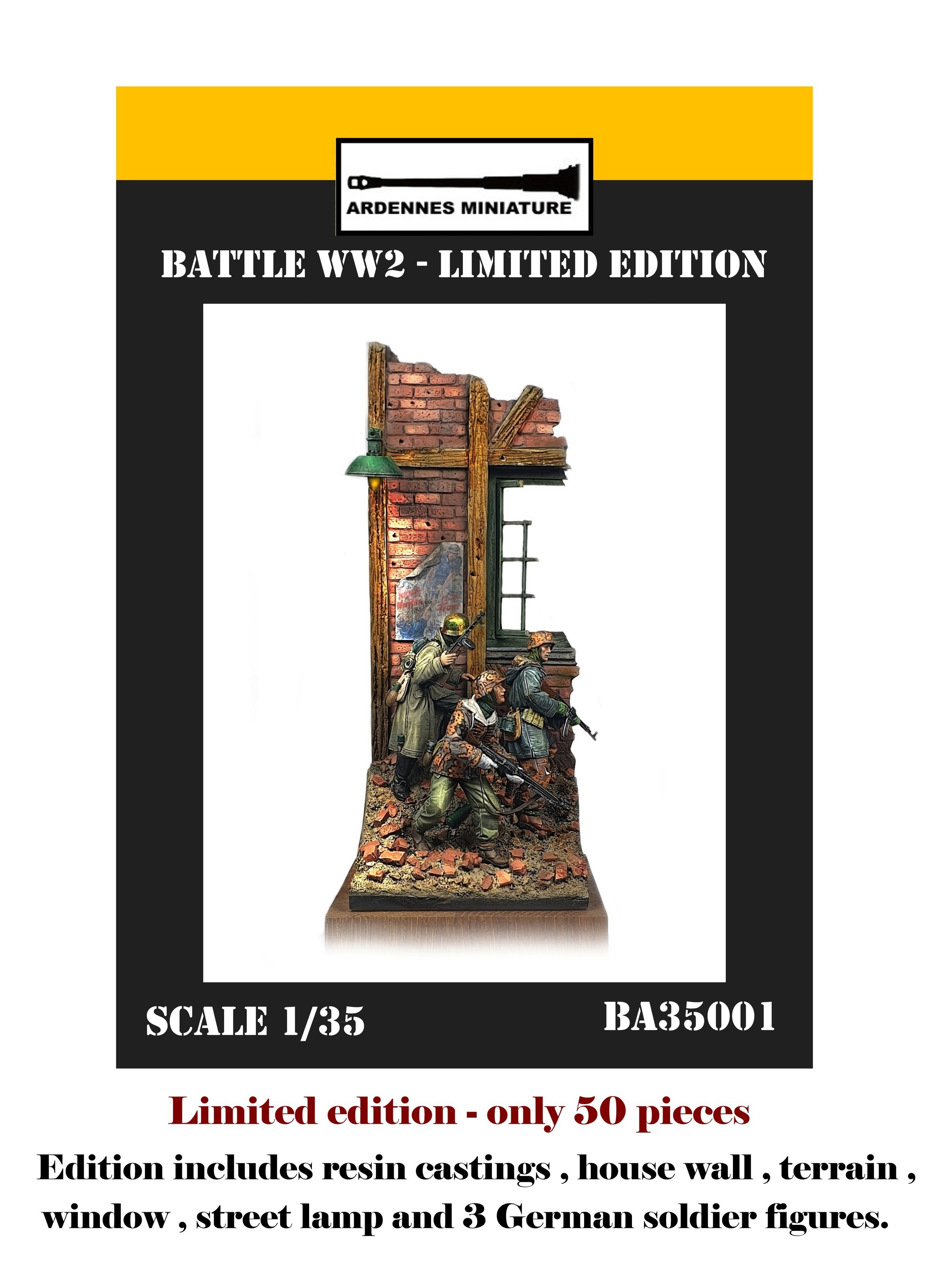This detailed close-up photo showcases an ad for a limited edition WWII memorabilia diorama titled "Ardennes Miniature, Battle WW2 Limited Edition." The diorama is presented against a white background with a black border and a goldish accent above. At the top of the ad, the title is prominently displayed in white lettering within the black border. Below, the imagery depicts a battle-scarred scene with three German soldiers wearing trench coats and combat fatigue pants, hunched down and hiding behind a heavily damaged brick wall. They are equipped with various assault rifles and appear to be sneaking and looking towards the right. The ground is strewn with broken red bricks and wooden beams, and a green desk lamp dimly lights the scene. A partially torn poster and a shattered window add to the war-torn atmosphere. At the bottom left of the ad, it specifies, "Scale 1:35, BA 35001, Limited Edition, only 50 pieces." It further details that the edition includes resin castings of the house wall, terrain, window, street lamp, and three German soldier figures. The background of the ad features black and goldish colors, enhancing the overall dramatic effect.